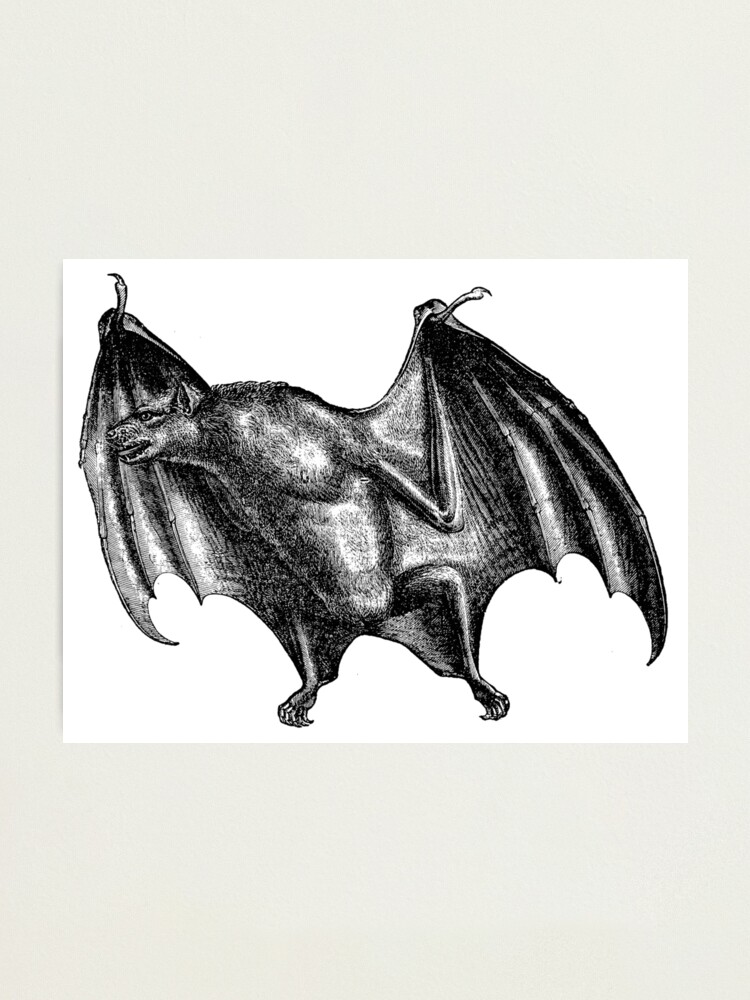The image presents a highly detailed, hand-drawn illustration of a bat set against a white rectangular card with a tannish, rectangular background. The bat, rendered in black and white, appears to be drawn with charcoal or pencil, featuring nuanced streaks and shading. The bat occupies the majority of the card, its fur, visible talons, and sharp teeth meticulously illustrated. The creature stands on its two legs with semi-outstretched wings, exposing its stomach, and is oriented towards the left side of the image. Its ears are prominently extended, and the drawing exudes a sense of hostility. A subtle, small cast shadow is visible to the left of the card, further accentuating the depth and intricacy of the artwork.